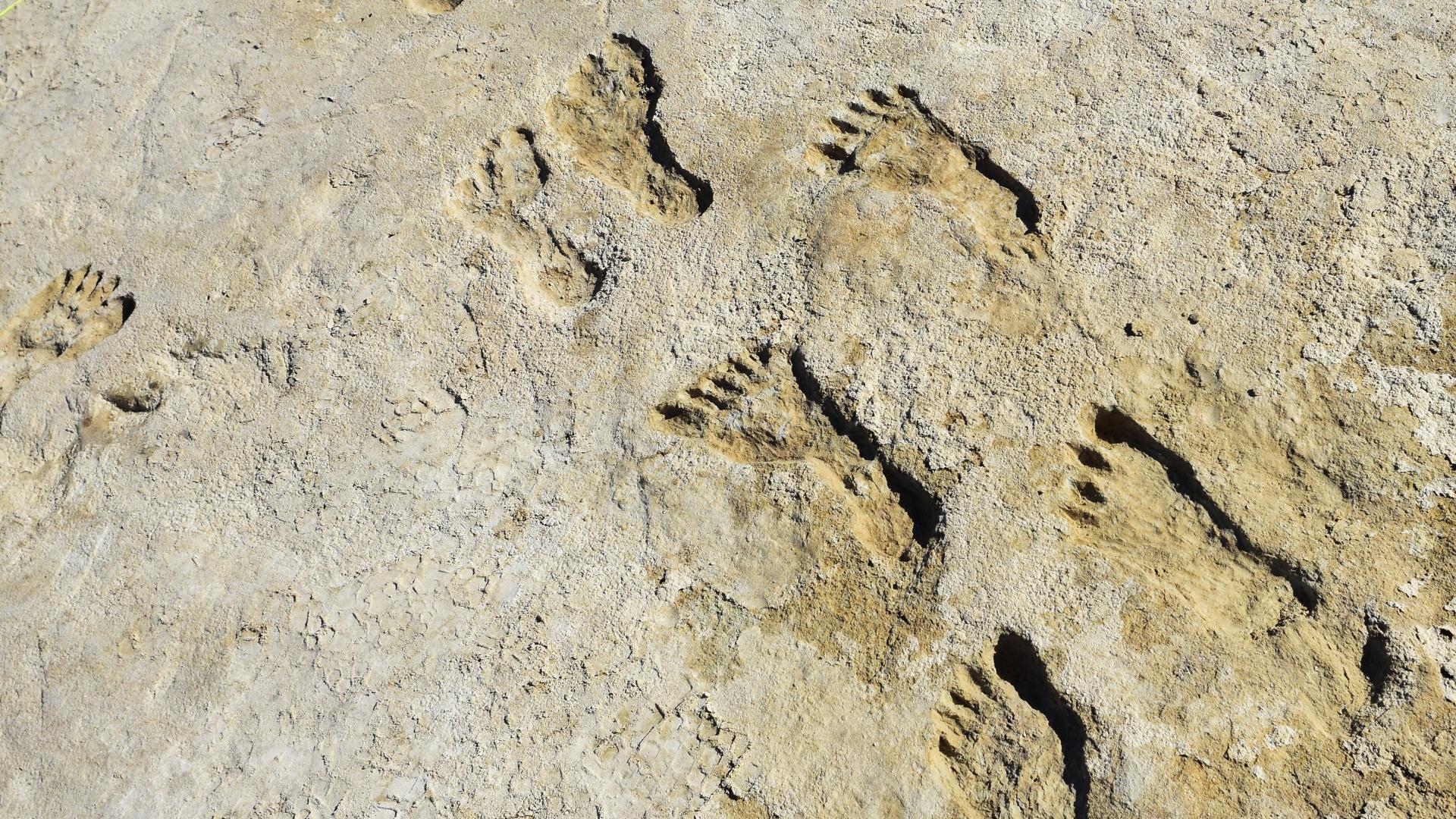The image captures a close-up view of a rocky surface with distinct imprints resembling various sets of footprints and possibly a handprint or an animal paw print. The rocky surface appears grayish with layers, possibly muddy at the top, and exhibits patches of tan, dark tan, brown, and black. There are three main sets of humanoid footprints, ranging in size and shape, with noticeable details like differently shaped toes and varying widths in the arches. The foremost set of footprints stretches from the bottom right towards the upper center of the image, overlapping each other. To the left edge, there is an imprint that could be either a hand or a foot. The positioning and formation of the prints suggest they were captured from an above angle, blended within the rocky, possibly fossilized or hardened terrain. The overall setting implies an outdoor environment, showcasing impressions that evoke fossilized remains emerging from the rock surface.